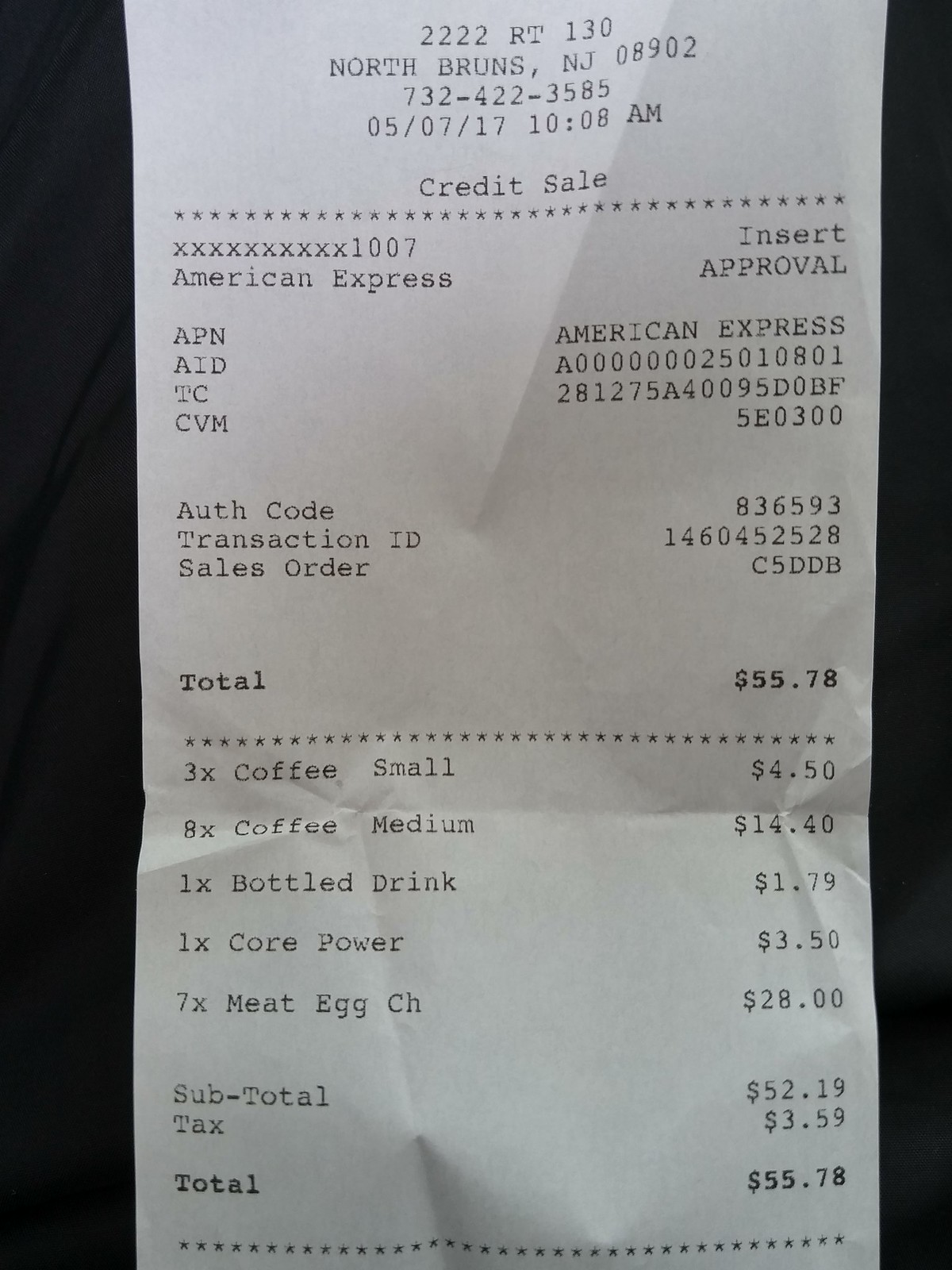This detailed image is a vertical photograph or scan of a receipt, likely taken with a regular camera. The receipt itself is printed on standard white receipt paper with black ink. The image features vertical black bars on both the left and right sides, suggesting the receipt is lying on a black background or table surface. 

At the top of the receipt, the store's information is listed: "222 RT 130, North Brunswick, NJ 08902," followed by the phone number "732-422-3585." The date of the transaction is "05/07/17," and the time is "10:08 a.m." Below this, the receipt specifies "credit sale," and a row of stars or asterisks spans the width of the paper. The transaction was processed with an American Express card, indicated as approved. 

Further down, the receipt details the items purchased: three small coffees, eight medium coffees, one bottled drink, one Core Power drink, and seven meat egg chickens. The subtotal, tax, and the final total, which is $55.78, are also clearly itemized. Additional rows of stars and various transaction codes and authorization numbers are scattered through the receipt, culminating in the detailed listing of purchased items and their respective prices, leading to the final total.